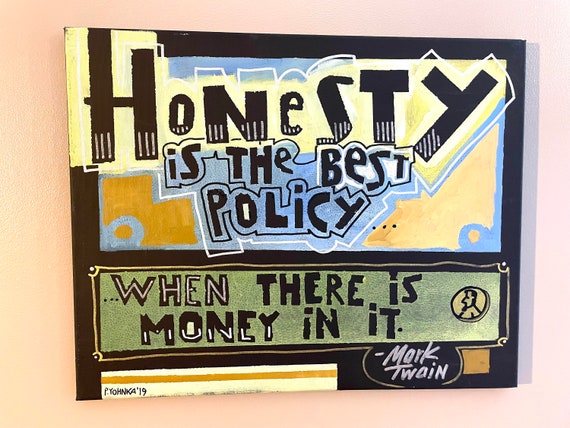The image depicts a vintage-style metal sign mounted on a tan-colored wall. The sign has a black border framing a central message that reads, "Honesty is the best policy," written in black text against a yellowish background. Above the word "honesty," there is a touch of blue, while below, the backdrop transitions into a blue hue. Towards the bottom of the sign, a green box with a blue background features the phrase, "when there is money in it," also in black text. Accompanying this text is a cartoon illustration of a penny bearing Abe Lincoln’s profile facing left. Below the penny, a black circle contains the word "Twain" in white text, attributing this sarcastic quotation to Mark Twain. Additionally, on the bottom left corner, there is a yellow rectangular box with a darker yellow stripe displaying the name "P-Y-O-H-N-K-A" followed by "-19". The overall design emphasizes a satirical twist on the famous saying, "Honesty is the best policy," by adding, "when there is money in it," highlighting the quote’s humorous and cynical undertone.